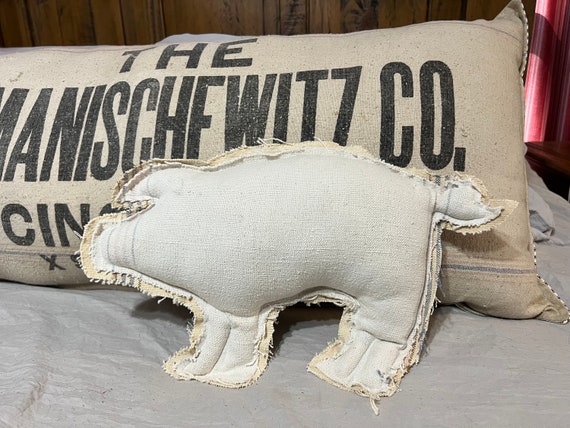The photograph depicts a zoomed-in section of a bed adorned with two pillows. The backdrop features wood paneling, suggesting it might be a bedroom, and faint light filtering through curtains in the far right corner of the image. The bed itself is covered in canvas-like bedding. Resting prominently on the bed is a long rectangular pillow that resembles a burlap or canvas sack, with black writing partially visible, indicating "The Manischewitz Co." and a partially obscured location hinting at "Cincinnati." This pillow is designed to mimic a feed sack. In front of it, there is an off-white, pig-shaped pillow with frayed, stringy edges, appearing roughly sewn and raggedy, adding a rustic charm to the composition.